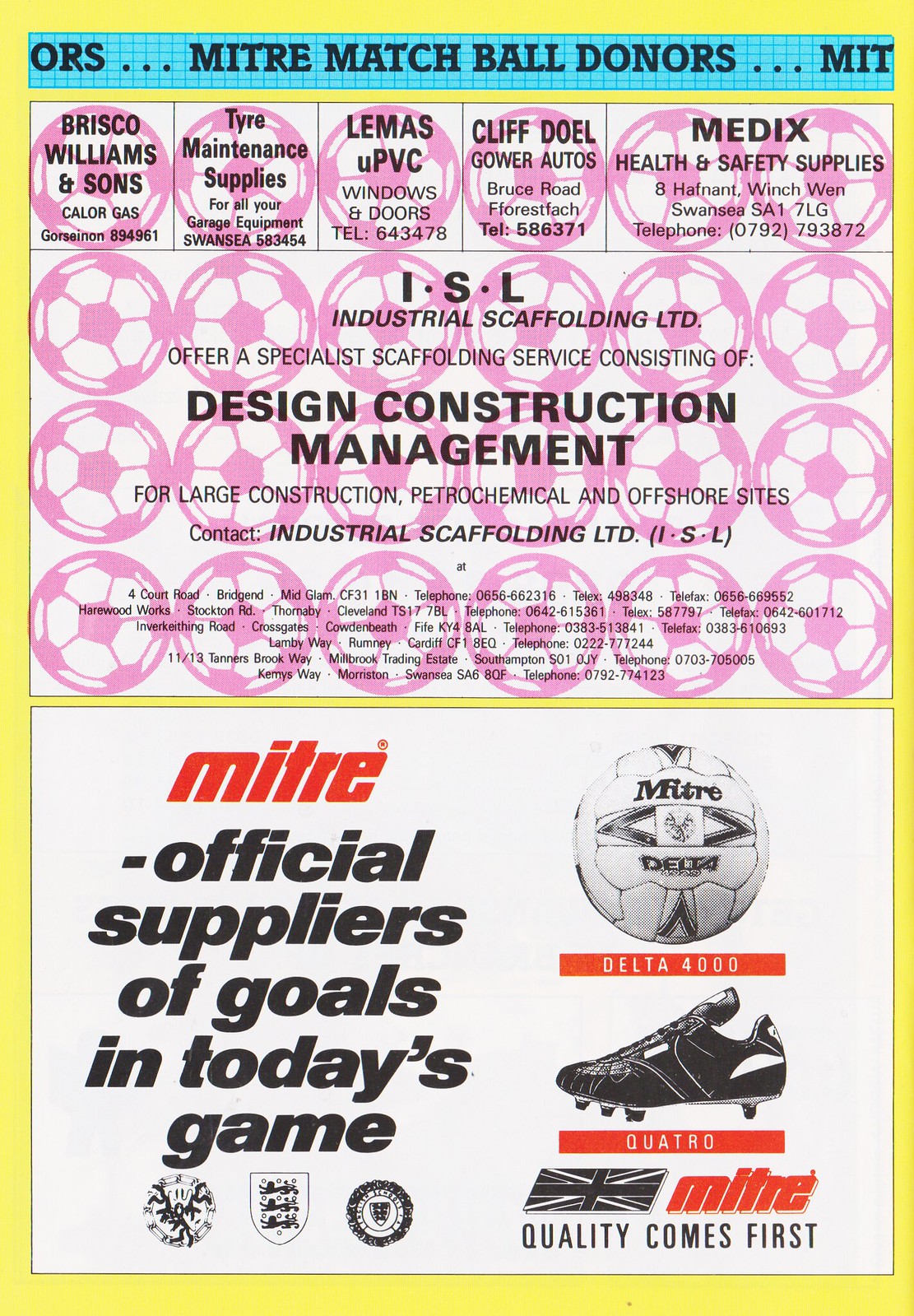This advertisement page is dedicated to highlighting sponsors of a soccer event. At the top, a blue banner with black uppercase font reads "MITRE Match Ball Donors." Below this banner, a row features five squares, each displaying different sponsor advertisements: Briscoe, William and Sons, Caller Gas, Tire Maintenance Supplies, LaMasse UPVC Windows and Doors, Cliff Dole Gower Autos, and Medix Health and Safety Supplies. Dominating a substantial portion of the frame is a large advertisement for Industrial Scaffolding Limited (ISL), emphasizing their expertise in design, construction, and management with extensive details about their services. The bottom half showcases "MITRE Official Suppliers of Goals in Today's Game," featuring a photograph of a soccer ball and an athletic shoe, underlining Mitre's commitment to quality in their products with the slogan "Quality Comes First" in red and black lettering. This collaborative sponsorship display underscores the businesses' support and association with the soccer game, leveraging the event for mutual promotion.